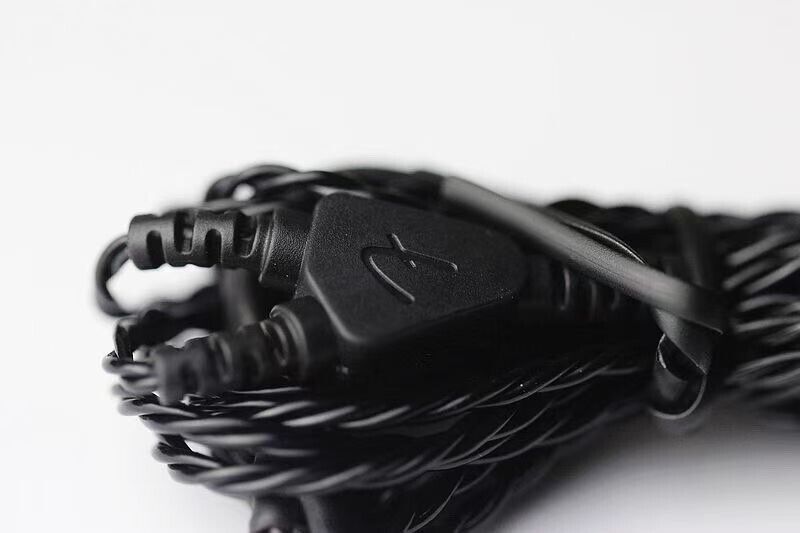The image is a black-and-white, close-up photograph showcasing a bundle of black cables against a light gray to white background. At the center of the frame is a prominent, upside-down triangular plastic connector, rotated so that its top points to the left. This connector features an engraved logo resembling the Fender guitar logo, which appears as a stylized, backward, lowercase 'f' or a seven-like symbol. Emerging from the left side of the connector are two slightly bent cylindrical extensions with alternating indents, from which dual black cables twist together, leading into a coiled mass of cables. This central bundle is cinched with a flat black cable, while other parts of the cables extend out of the frame to the right. Due to the shallow depth of field, the edges of the cables blur, drawing focus to the detailed connector and its engraved symbol.